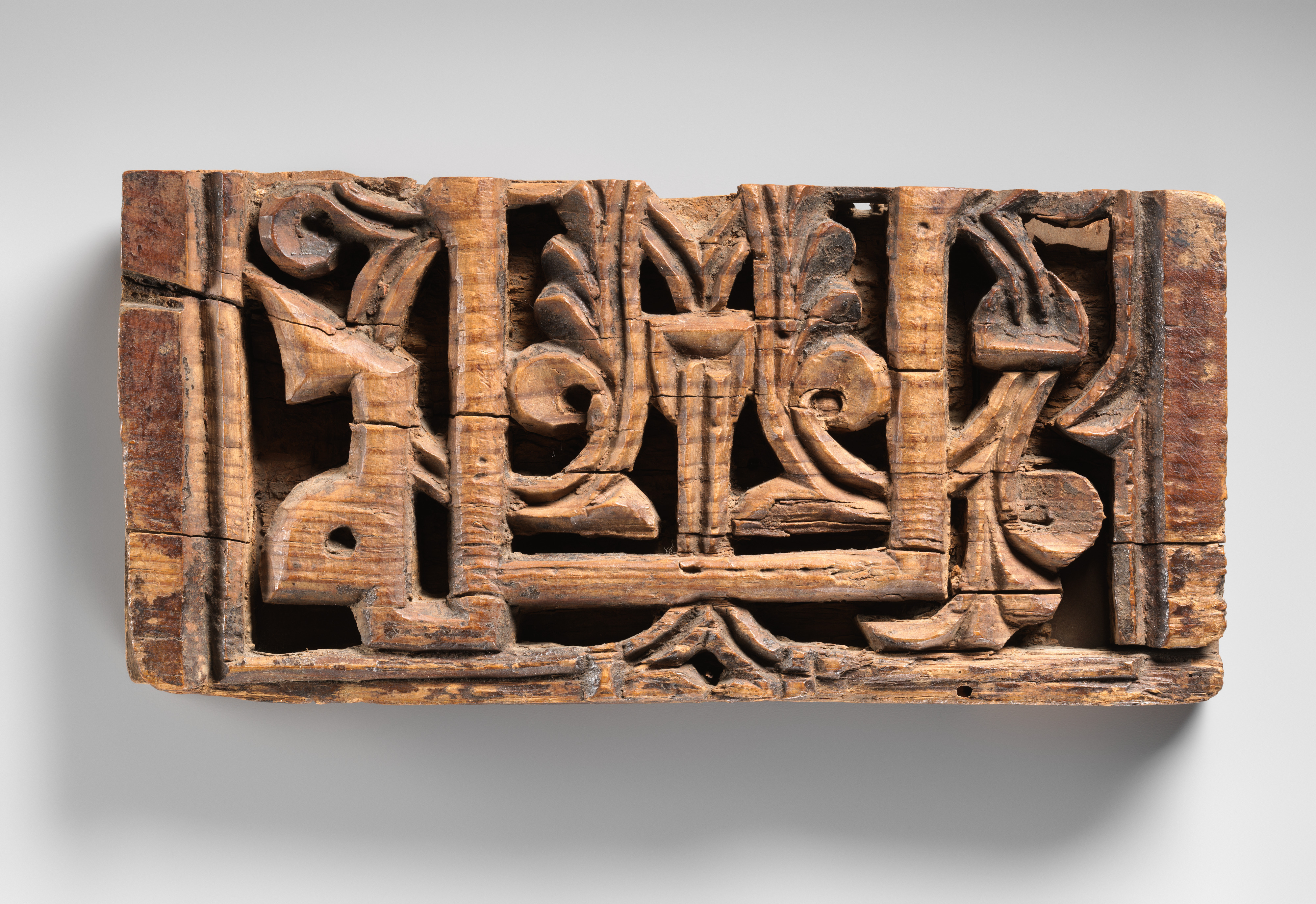This color photograph features a rectangular piece of intricately carved brown wood, likely an antique artifact, resting against a plain white background. Measuring approximately seven to eight inches in length and three to four inches in width, the wood appears aged, with visible cracks and a somewhat dry texture. The central design is quite detailed, depicting an abstract figure that resembles a person with a triangular headdress, formed by a V-shaped head and an upside-down U for the shoulders, with two long lines extending down as legs. Surrounding this figure, the carvings include wave-like patterns at the bottom and leaf-like shapes on both sides, enclosed within a box-like frame that leaves the top open. Additional abstract elements, like a reversed lowercase 'd' and plant-like forms, are also present within distinct, walled-off sections. The wood around these central designs appears to have been lightly sanded but retains a rustic, somewhat unfinished look.